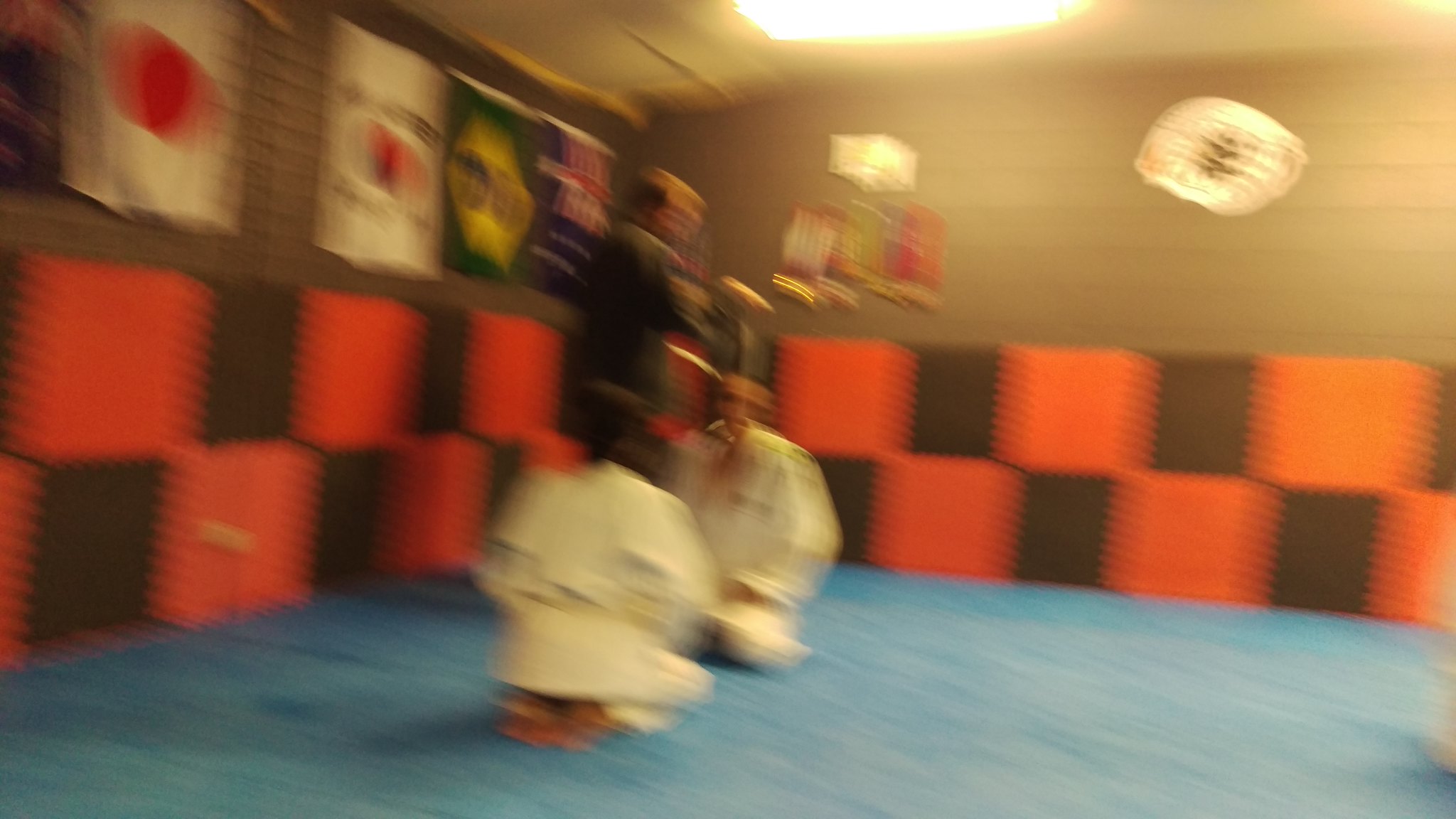The image is a very blurry photograph taken from a first-person point of view inside a karate dojo. The dojo features gray walls lined with a checkerboard pattern of black and red exercise mats, stacked in two rows around the entire room. These mats are approximately a foot and a half square each. The floor is covered with blue carpet. 

On the left wall, several flags hang, including a clearly identifiable Japanese flag. Other flags are difficult to discern due to the blur, but potential candidates mentioned include those of Korea, Brazil, Australia, and the Philippines. 

In the center of the image, two individuals wearing white robes and kneeling on the floor face each other, positioning their hands and fists on their thighs. A man in a black robe, possibly a sensei or coach, stands over them with his hands in motion near one of the kneeling individuals, who appears to have dark hair tied into a bun or ponytail. The dojo is illuminated by a large fluorescent light fixture in the ceiling, positioned centrally in the image.